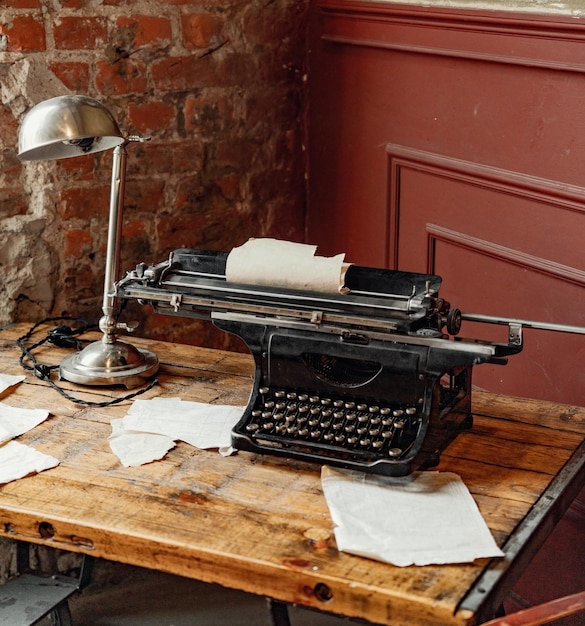The photograph showcases a well-used, vintage black mechanical typewriter perched on an aged, paneled wooden desk. The wood is worn, bearing stains that speak to its extensive use. The desk features a gray metal strip on the right side and is strewn with papers, some torn, suggesting a writer’s frustration or hurried composition. A sheet of paper sits in the typewriter, ready for more words to be hammered out by its individual mechanical keys. Just to the left of the typewriter is a brass lamp with a round base and a thin, circular neck leading up to a bulb attachment, illuminating the workspace. The background consists of a reddish-brown paneled wall behind the typewriter, while to the left, an old brick wall with weathered marks adds to the room’s antiquated charm. The scene exudes an atmosphere of literary endeavor within a space that has seen many years of creative toil.